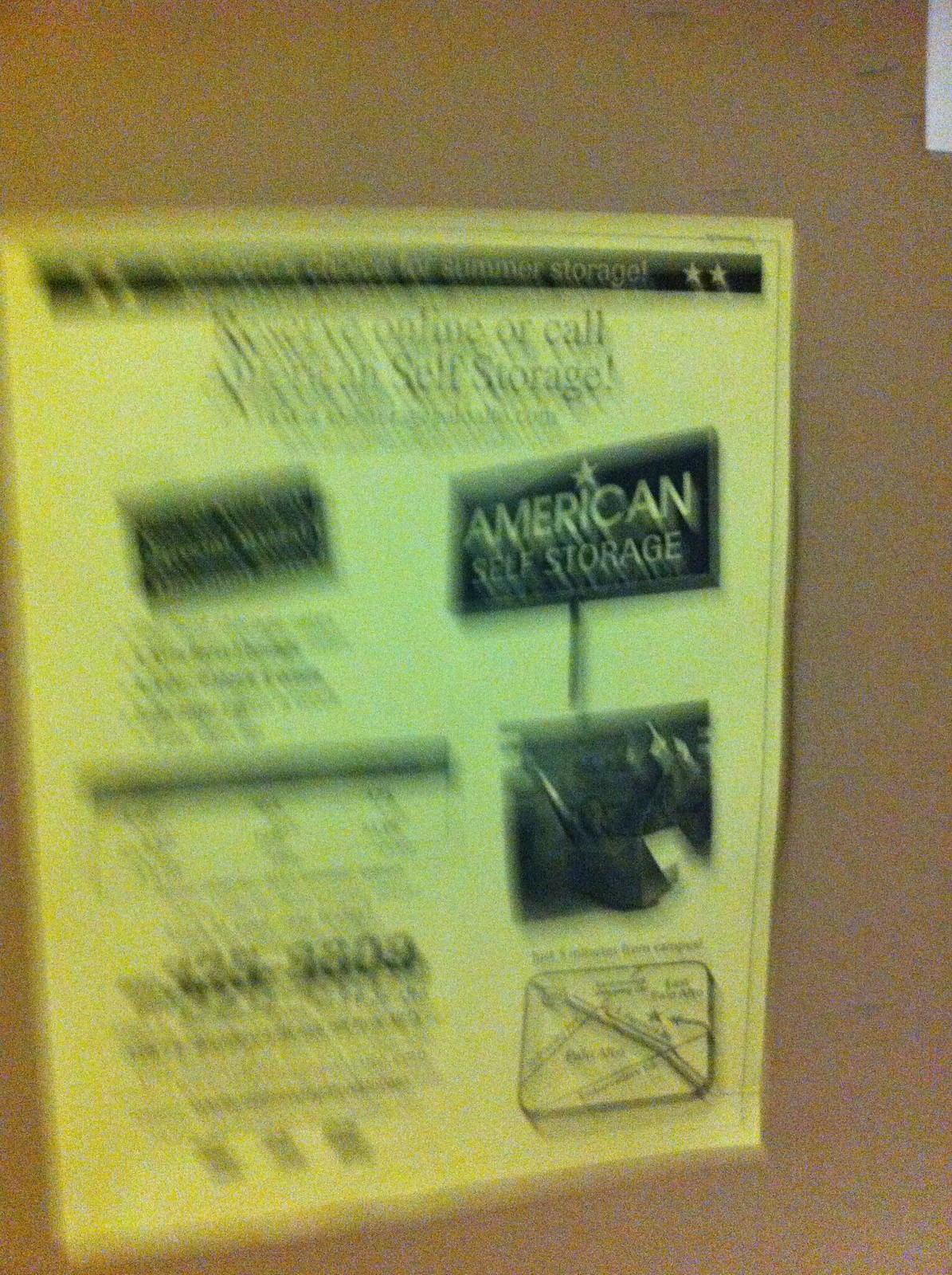This color photograph captures a yellow poster mounted on a beige wall, although the image is quite blurry and out of focus. The poster prominently features large black graphics at the top, including a black strip that spans the width. Below this strip, there are two lines of text that are difficult to decipher due to the blur, but the word "self-storage" is barely legible. Towards the middle-right area of the poster, the company's logo is partially visible; it reads "American Self-Storage" in yellow text set against a black rectangular background. Below this, a black square likely contains additional writing, though it’s indistinct. Similarly, the left side of the poster has extensive text, but none of it can be read clearly due to the lack of focus.